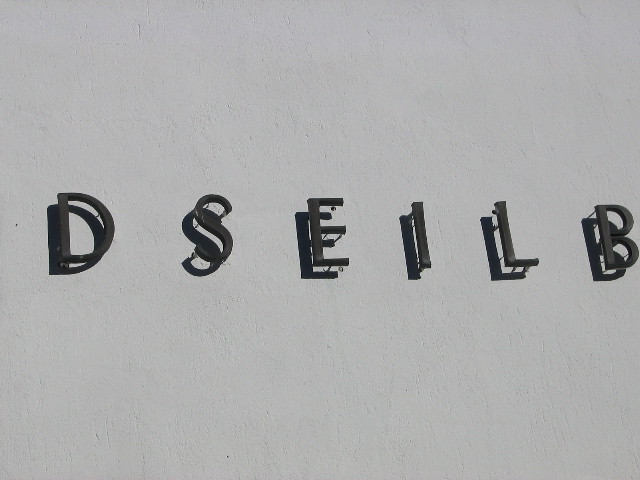The image is a color photograph taken outdoors, showcasing a textured plaster wall with slight imperfections and discoloration. The plaster is an off-white shade with subtle undertones of light brown, adding a slightly cream appearance. Raised black letters mounted on the wall are attached with small black poles, creating distinct shadows behind them. The sunlight seems to originate from a position slightly behind and to the right of the viewer, at an approximate 45-degree angle, casting the shadows to the left and slightly downward. The visible letters in the photograph are "D," "S," "E," "I," "L," and "B," though the image is cropped closely and the context suggests there could be more letters extending beyond the right edge. The letters themselves appear to be made of wrought iron, adding a touch of elegance and durability to the scene.